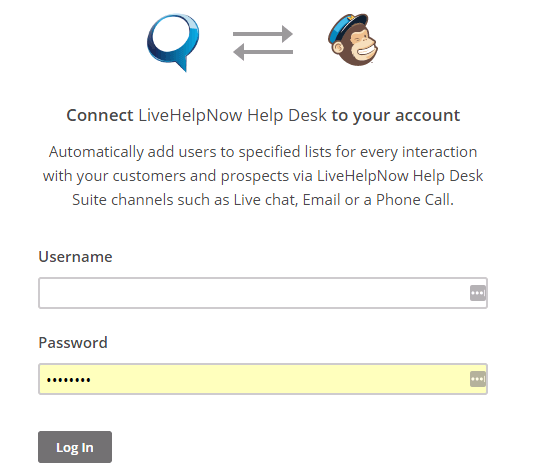In this help page image, the layout is as follows: At the top, there is a blue circle with a curved arrow inside it. Next to the circle, an arrow points towards a symbol depicting a monkey wearing a blue hat, which then has an arrow pointing back to the blue circle below it. 

The page headline reads "Connect," written in a bold font, followed by "Live Help Now Help Desk to your account," with "to your account" emphasized in even bolder text. Below this headline, a description in gray letters states, "Automatically add users to specified lists for every interaction with your customers and prospects via Live Help Now Help Desk. Sweet channels such as live chat, email, or a phone call."

Further down the page, there is a form starting with the label "Username" in black letters, followed by a blank white input rectangle. Below this, the form label "Password" is also written in black letters with a filled yellow rectangle where the password is entered, represented as dots for security.

At the bottom-left corner of the form is a small gray button with the word "Login" written in white letters.